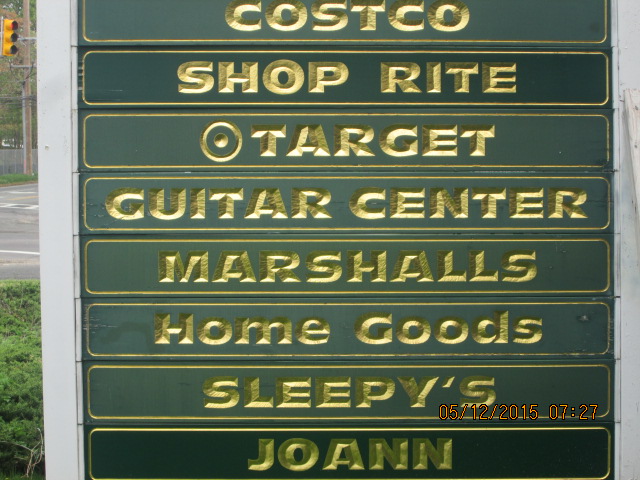The photograph captures a sign positioned outside a large shopping center, prominently listing the stores within it. The sign is constructed with two upright wooden posts supporting green wooden slats, each meticulously routed with the name of a store and painted in a vibrant yellow. From top to bottom, the stores listed are: Costco, ShopRite, Target, Guitar Center, Marshalls, Home Goods, Sleepy's, and Joanne. A timestamp in the lower right corner of the image reads "05-12-2015 at 7:27." While the sign dominates most of the frame, a narrow strip on the left reveals a patch of grass, the intersecting asphalt roads, and a side view of a traffic light, situating the scene in a suburban setting.